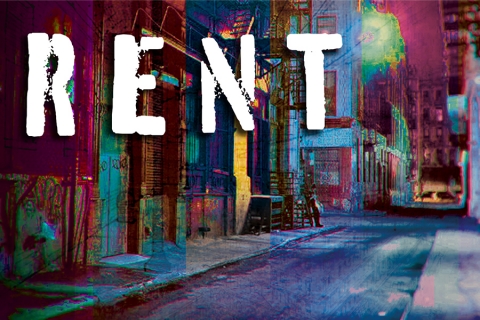This vibrant, colorized image—likely a poster or advertisement for the Broadway musical "Rent"—features the word "RENT" prominently in large, stenciled white letters in the upper left-hand corner. The scene appears to be an enhanced photograph or artwork depicting an alleyway or city street, probably set in New York City at nighttime. The background showcases a kaleidoscope of buildings in various colors such as purple, brown, turquoise, green, indigo, dark purple, and yellow, all contributing to a random, almost painted-on aesthetic. 

A dark blue road splits into two directions and runs through the center of the image, flanked by colorful buildings that stretch into the distance. Fire escapes and a street lamp enhance the urban atmosphere. Although the scene is rich with architectural details, it appears desolate, with no people or motor vehicles present, except for a possible figure leaning against a fire escape. This wide-format image captures the eclectic, gritty essence of the city, setting an evocative tone for the musical it advertises.